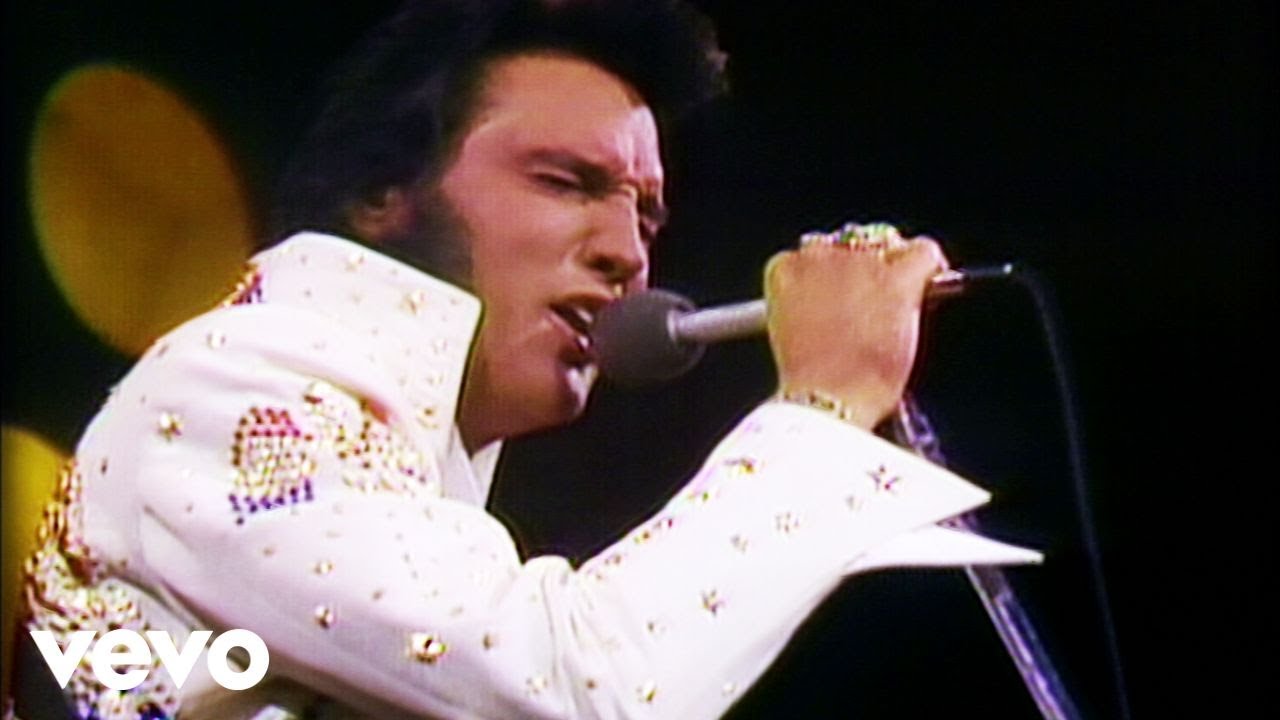The photograph captures Elvis Presley in an intense performance. Positioned centrally from the right side, Elvis is dressed in an iconic white sequined jumpsuit adorned with intricate purple, red, and golden patterns. His right arm is raised, gripping a microphone, while several gold rings glint on his fingers. His eyes are closed, deeply immersed in his singing. The black background starkly contrasts with a couple of dim, yellow circular lights on the left. In the bottom left corner, a white watermark stipulates "Vivo," suggesting a possible YouTube thumbnail from a vintage, low-resolution recording.